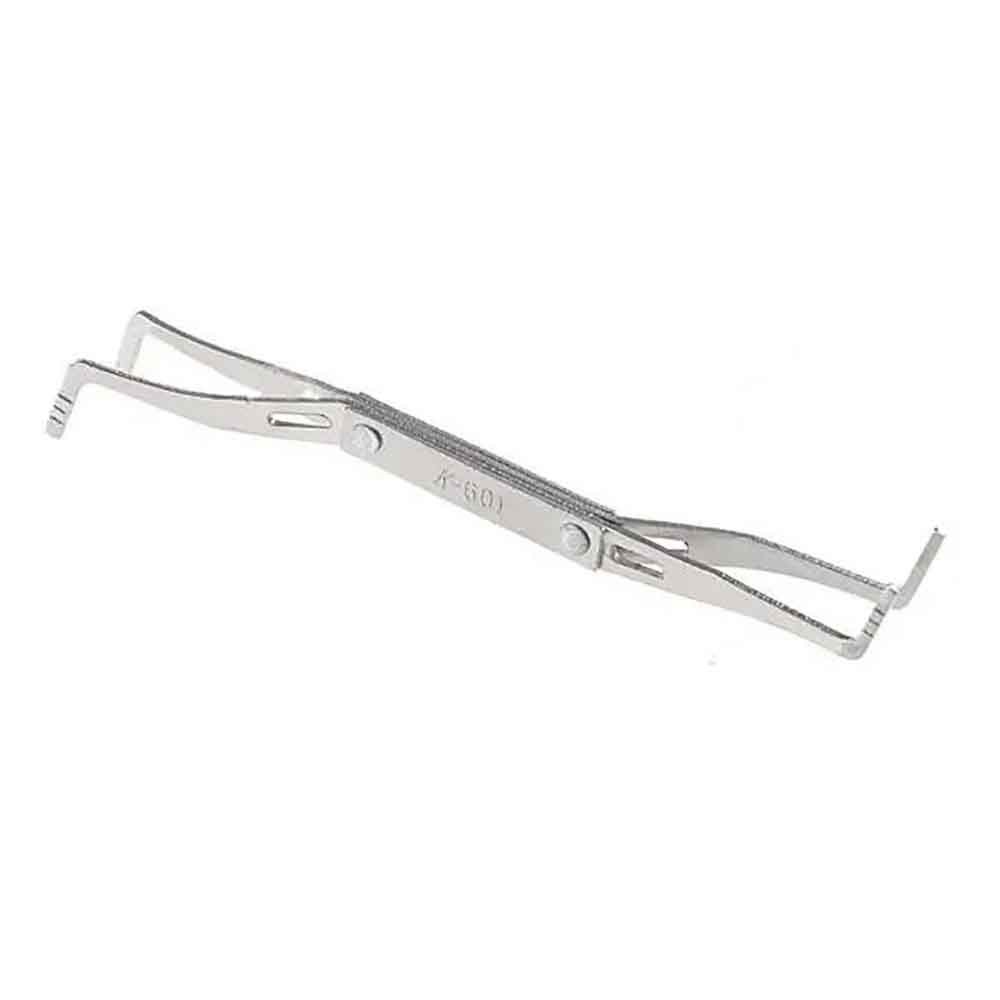The image depicts a double-ended stainless steel tool, resembling tweezers or forceps, measuring approximately eight inches in length. One end features prongs that face upward, while the opposite end has prongs facing downward, each about an inch long. The tool is designed with a flat, thin handle at the center, which bears an engraving marked "K-601." The prongs on both ends are equipped with three small dashes each. The tool, possibly used in surgical or scientific applications, is photographed against a completely white background, providing no additional context or labels regarding its specific use.